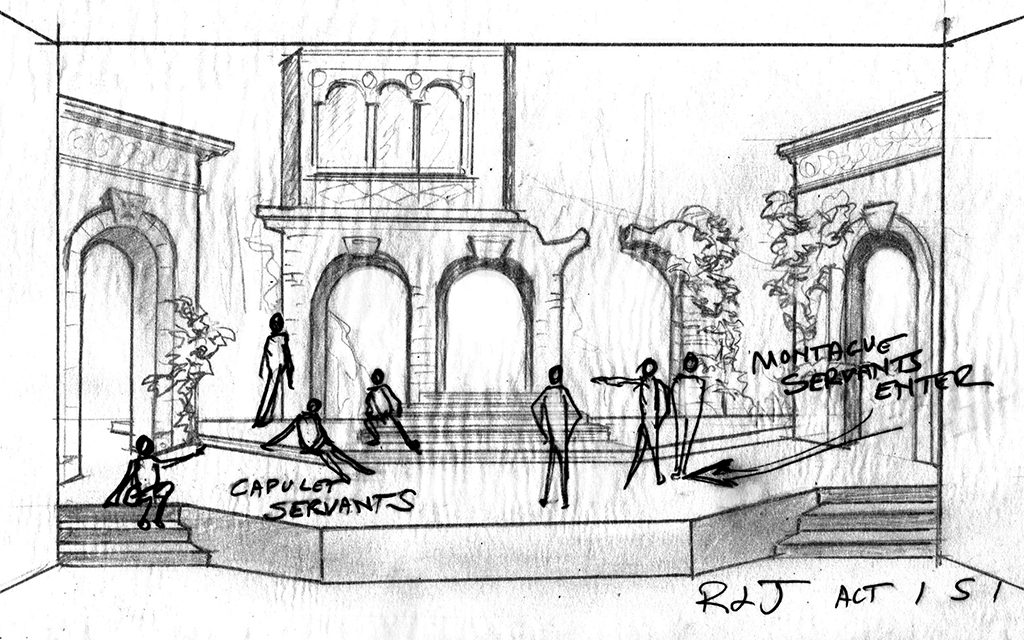This detailed hand-drawn illustration appears to be a vintage sketch for a stage production of Shakespeare's "Romeo and Juliet," specifically Act 1, Scene 1. The scene depicts a set that includes ancient, ruined buildings with arched entryways and vines climbing the walls, reminiscent of old Italy. The stage features steps on either side, each with three steps leading to the main platform and the background buildings.

In the lower right corner, the sketch is annotated with "R&J Act 1 Scene 1." Throughout the illustration, there are figures drawn in two distinct styles: the stage and buildings are crafted in lighter, pencil strokes, while the characters are depicted in darker, more defined lines, suggesting a different artist added them later using a felt pen or ink gel pen.

To the left, four darker figures are positioned on the stairs with a label beneath them reading "Capulet Servants." On the right, three more figures are annotated with "Montague Servants Enter," accompanied by an arrow indicating their movement. These details provide a sense of the staging directions for the scene, making the sketch a valuable reference for the production's layout and actor positioning.